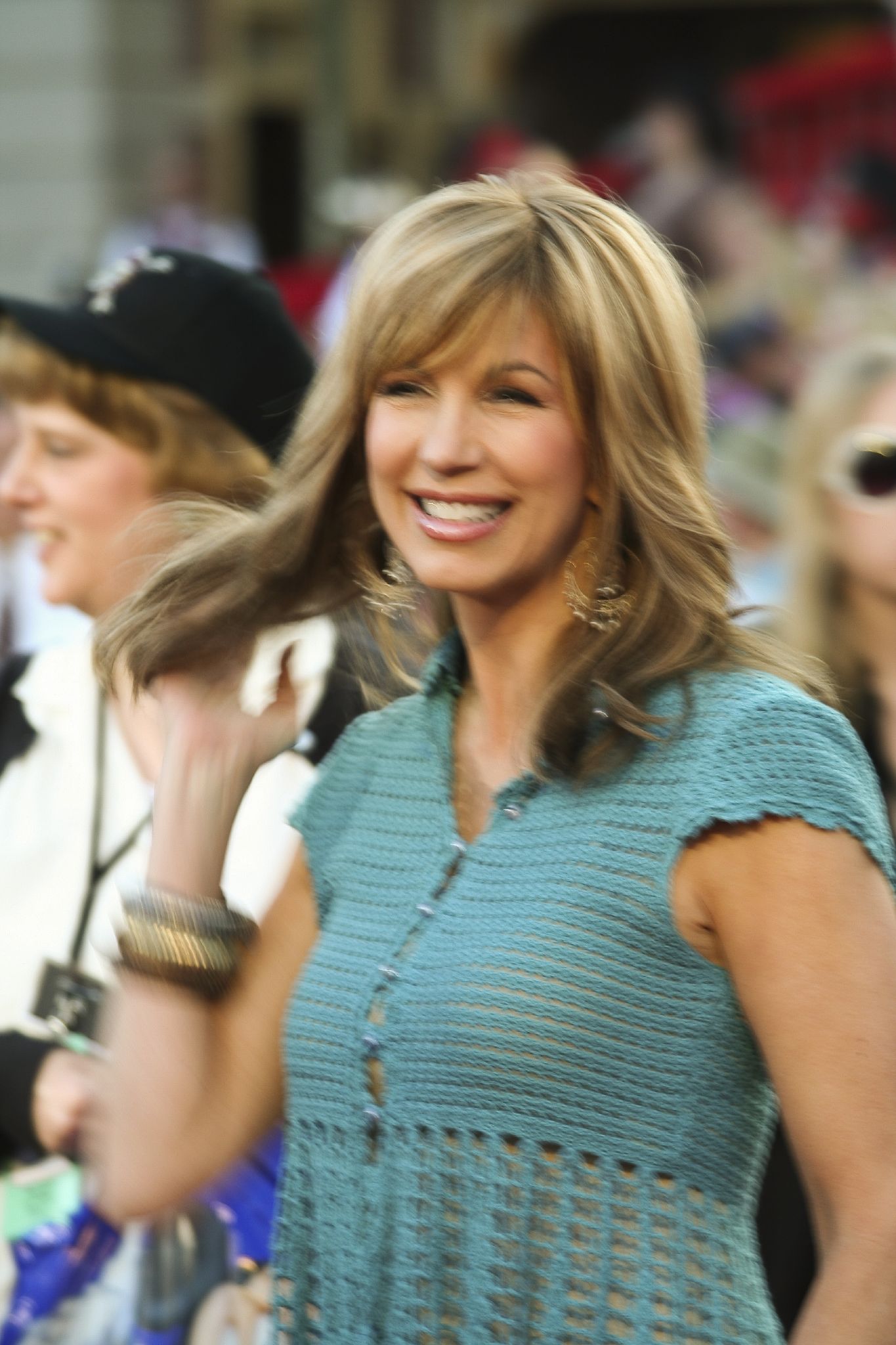In this slightly out-of-focus photograph, Lisa Gibbons is prominently featured from the waist up, standing amidst an out-of-focus crowd at what appears to be a sporting event. Lisa, who is smiling, is flipping her hair with her right hand. She has long, blonde-highlighted hair that just reaches her shoulders, with bangs framing her face. She is adorned with large, ornate gold chandelier earrings and multiple chunky bangles on her right arm. Lisa is dressed in a seafoam green, short-sleeved knit blouse that includes cap sleeves, a button placket up the center, and intricate weave patterns—tighter across the chest and more open like netting below the bust.

In the background, we can make out several spectators, one of whom is particularly noticeable over Lisa's left shoulder. This individual is a woman with reddish-brown hair, wearing a black baseball cap, white shirt, and black lanyard with a bag attached. Other colors present in the image include teal, white, black, royal blue, red, purple, brown, and tan. The diverse hues and indistinct forms suggest a vibrant, outdoor daytime setting focused entirely on Lisa Gibbons as she revels in the moment.